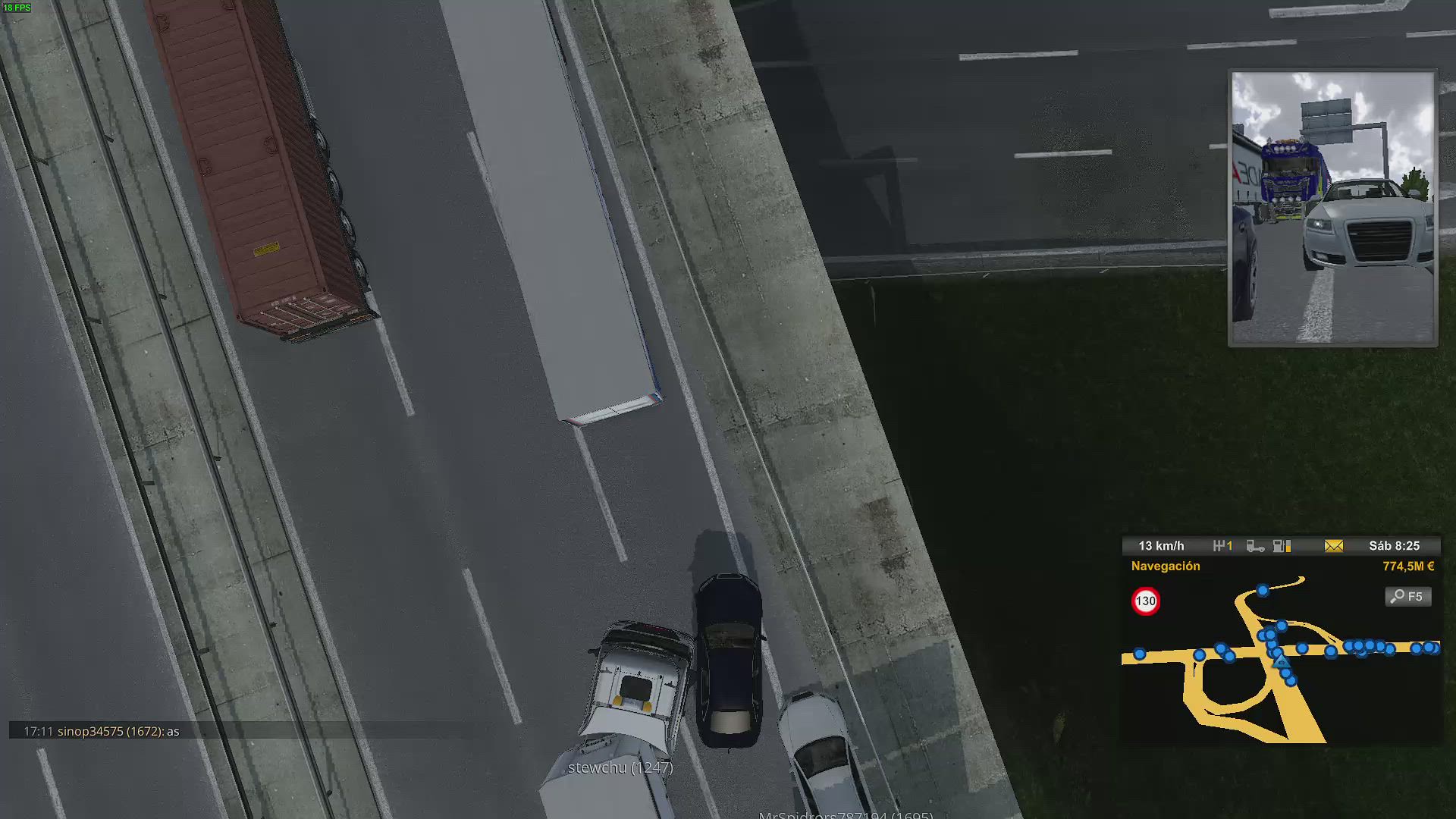The image, a color landscape-style piece that appears to be computer or AI-generated, captures an aerial perspective of a highway scene dominated by gray and black hues. The highway, starting at the bottom of the illustration and tilting upwards to the left, features several vehicles. A long white truck and a long dark brown truck are seen from the top, traversing the road. At the image's bottom, a small gray car and a small black car, which is slightly tilted to the right, are present. The white truck's cab is depicted colliding with the black car from the left side. Additionally, the image includes two insets: one shows a white car from a head-on view, while the other displays a map marked with blue circles.